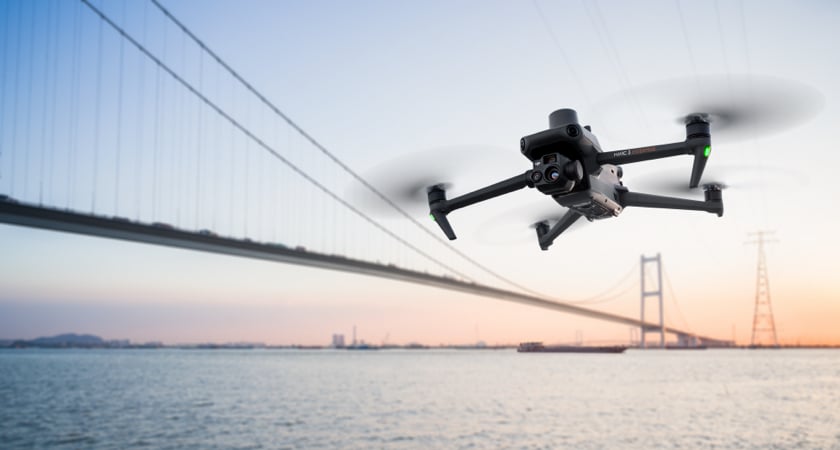A detailed photograph captures a black quadrotor drone in flight, hovering in the foreground with all four rotors spinning and a green light indicating it's possibly recording. The scene is set against the iconic San Francisco Bay Area backdrop, with an extremely long cable suspension bridge stretching across the water. This bridge, potentially the Golden Gate Bridge, leads towards a distant cityscape shrouded in the softened hues of either early morning or late evening light, as suggested by the light blue sky transitioning to muted orange near the horizon. To the left of the frame stands a massive high-voltage electric tower, its wires crisscrossing the sky. The vast expanse of water beneath the bridge and the distant shoreline complete this picturesque blend of modern technology and natural beauty.